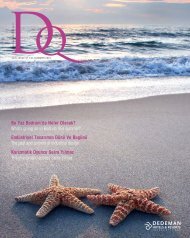The image is a small advertisement, possibly for travel, featuring a serene beach at sunset. In the foreground, two large and beautiful starfish, one darker than the other with white accents on their legs, rest on the smooth, untouched sand. The ocean, with its gentle waves, meets the horizon where the sky glows with hints of pinks and yellows from the setting sun. Puffy white clouds drift across the sky, adding to the peaceful ambiance. At the top left corner, "DQ" is prominently displayed in a magenta or purple font. Accompanying text in alternating lines of magenta and white, though largely unreadable due to its small size, hints at a connection to New Orleans. The bottom right corner contains the name "Dedeman" and a small icon, both in white. Overall, the image conveys a tranquil seaside scene with a touch of mystery in its messaging.